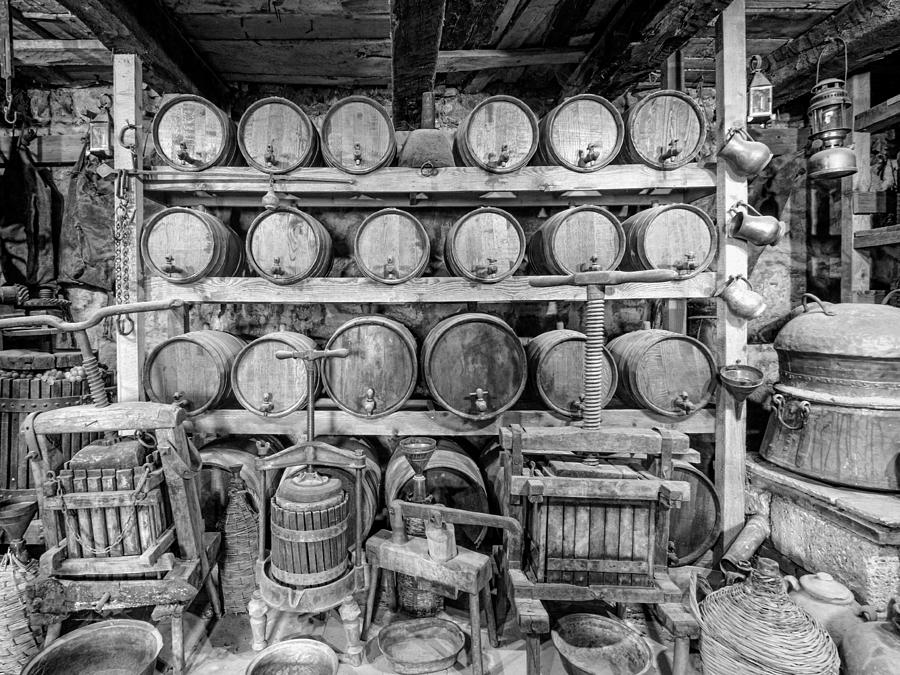This rectangular, black and white photograph depicts an old, rustic indoor scene, likely the interior of a vintage winery or distillery. The ceiling features exposed wooden beams, emphasizing the primitive and raw setting. Central to the image is a large wooden shelf stacked with numerous barrels oriented sideways, each equipped with a spigot or tap, suggesting their use for storing wine or other alcohol.

In the foreground, multiple pieces of vintage machinery are visible, including a grape-crushing device. This apparatus has a bucket with a plunger and a handlebar mechanism designed to press grapes, with a spout at the bottom draining into a pan. Another visible machine features a helical screw and handles that twist a large screw to crush grapes in a square box, also fitted with a draining spout and pan beneath.

Additionally, various cups with handles hang from a wooden pillar, and scattered around the scene are pots, pans, metal buckets, and other primitive tools and devices associated with winemaking and alcohol production. The wooden elements and mechanical equipment give the scene a historical atmosphere, capturing a moment frozen in time.